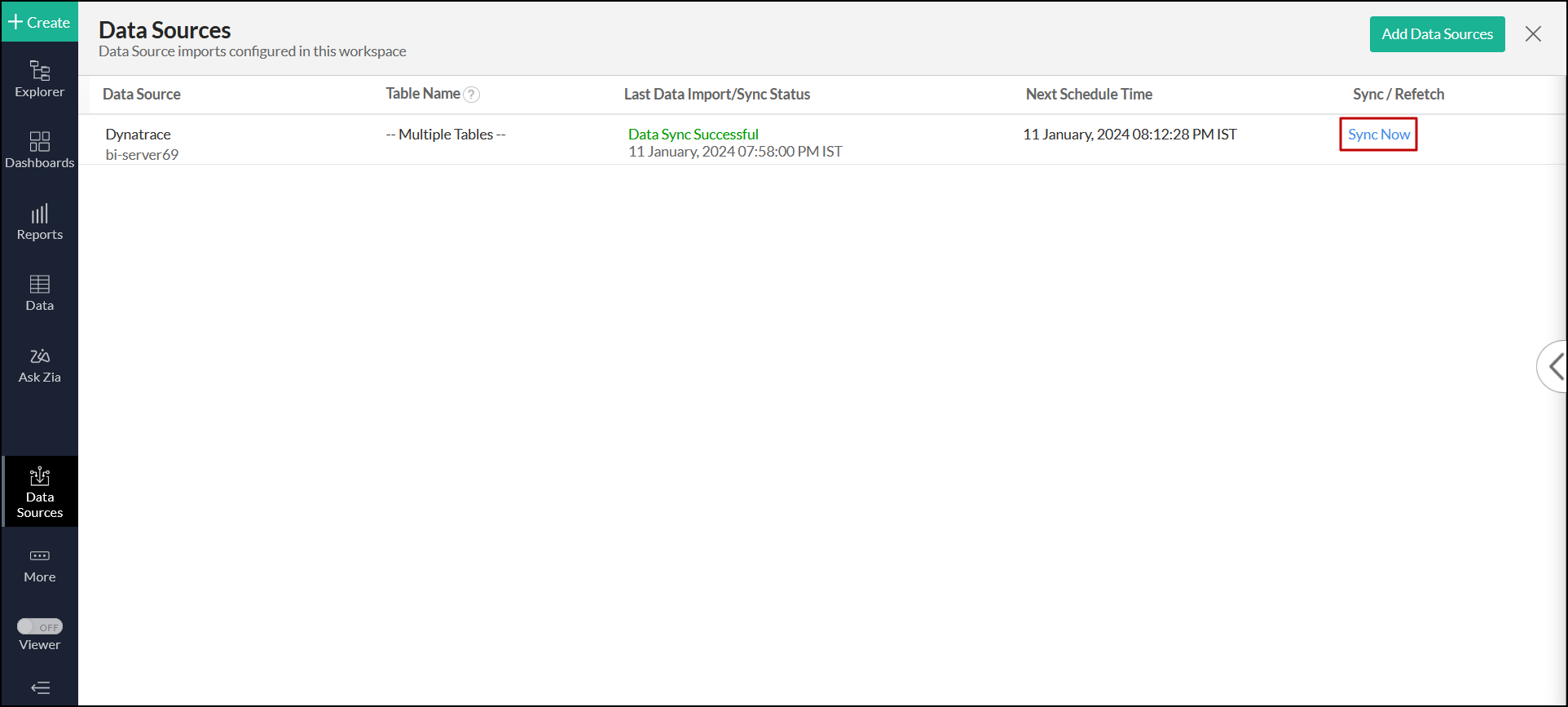The image depicts a diagram with a variety of colored rectangles and text of varying sizes. The main focus is a black-outlined large rectangle that encompasses several distinct areas.

At the top-left corner, there is a small green rectangle containing words and symbols, followed immediately below by a long blue rectangle with more words and symbols, though both sets of text are too small to read. Near the bottom of the blue rectangle, there is a black square featuring a symbol and some words, also difficult to discern. Below the black square, the blue rectangle continues with more text and symbols, followed by a bulging white rectangle on both its left and right sides, containing additional words and symbols.

Moving to the top of the diagram, spanning the entire width, is a light gray rectangle with the word "Dinosaurs" prominently displayed, accompanied by illegible smaller text beneath it. On the right-hand side of the diagram, another green rectangle is situated, also filled with unreadable text and marked by a gray "X."

Below this on the right side, there is a white rectangle that has a sequence of black words across the top, with successive lines of text in black, green, and black again. Finally, at the very bottom, a red-outlined rectangle contains a single word in blue, adding a distinct splash of color to the otherwise text-heavy diagram.